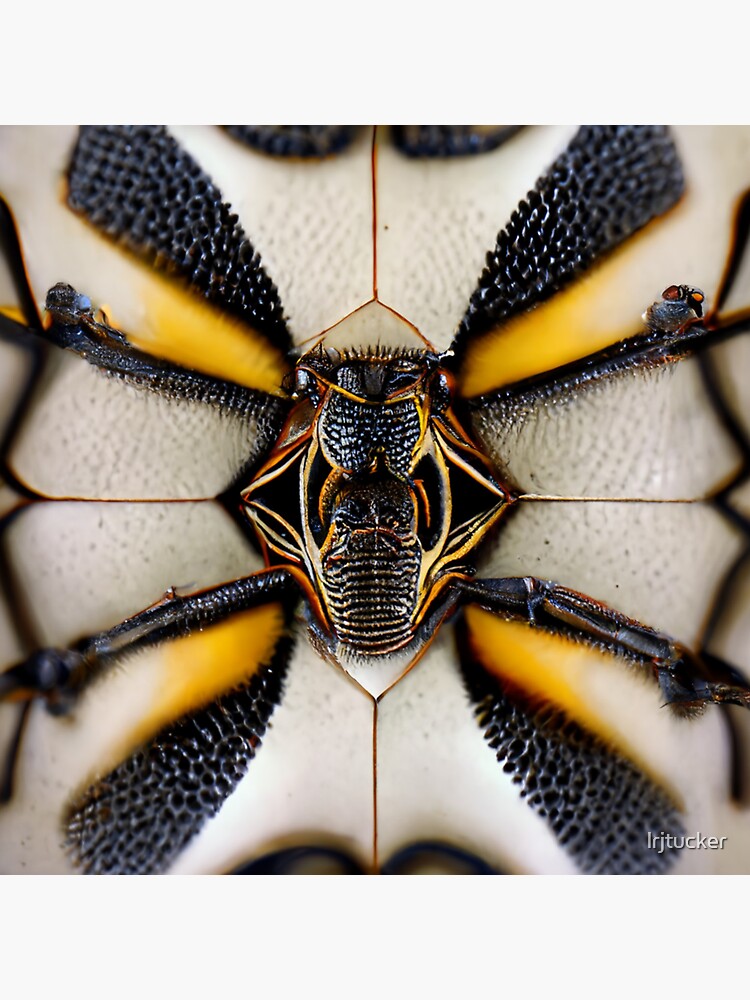This image captures a remarkably detailed, close-up view of an insect from its underside, with a symmetrical and vibrant coloration that includes whites, blacks, yellows, and oranges. The insect's spread wings display intricate patterns and lines, resembling stained glass with black and yellow stripes interwoven with yellow accents. The bug itself features a white body with a predominantly black torso highlighted by red and orange touches. Its eyes are prominent and centrally placed, giving an intense, almost anthropomorphic impression that the insect is staring at you. The legs or extenders into the wings are finely detailed, revealing tiny pricks. Overall, the image is focused sharply on the insect, with blurred edges enhancing the central view. In the bottom right corner, the watermark "LRJ Tucker" is visible, adding a professional touch to this realistic and vivid photograph.